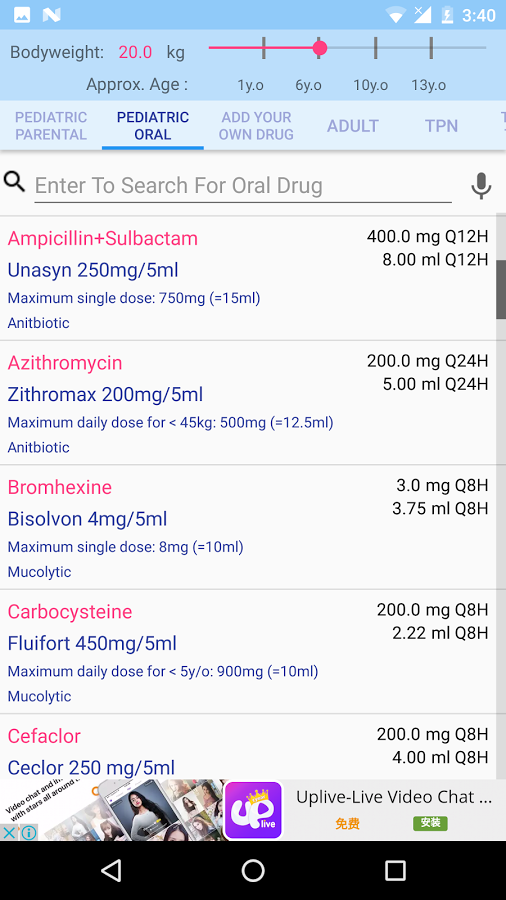**Detailed Caption: Pediatric Dosing Interface of a Medical Application**

This detailed screenshot showcases a pediatric dosing interface from a medical application, specifically designed for calculating oral drug dosages in children. 

**Overview:**
- **Patient Information:** The patient's body weight is prominently displayed in red text, reading **20 kilograms**. The child's approximate age is noted as **6 years old**. An adjustable **age slider** ranges from **1 year to 13 years**.
- **Tabs and Options:** The interface highlights the currently selected tab: **Pediatric Oral**. Additional tabs are available for **Pediatric Parenteral**, **Adult**, and **TPN** (Total Parenteral Nutrition).
- **Search Functionality:** A search bar labeled “**Enter to search for oral drug**” is accompanied by a search icon to facilitate drug searches.

**Drug Dosage Information:**
1. **Ampicillin plus Sulbactam (Unicin)**
   - **Strength:** 250 milligrams/5 milliliters
   - **Dosage:** 400 milligrams every 12 hours (400 mg/q12h)
   - **Volume:** 8.00 milliliters every 12 hours (8 ml/q12h)
   - **Maximum Single Dose:** 650 milligrams (15 milliliters)
   - **Category:** Antibiotic

2. **Azithromycin (Zithromax)**
   - **Strength:** 200 milligrams/5 milliliters
   - **Dosage:** 200 milligrams every 24 hours (200 mg/q24h)
   - **Volume:** 5.00 milliliters every 24 hours (5 ml/q24h)
   - **Maximum Dosage (for under 45 kilograms):** 500 milligrams (12.5 milliliters)
   - **Category:** Antibiotic

3. **Bromhexane (Bisloxetamine)**
   - **Strength:** 4 milligrams/5 milliliters
   - **Dosage:** 3 milligrams every 8 hours (3 mg/q8h)
   - **Volume:** 3.75 milliliters every 8 hours (3.75 ml/q8h)
   - **Maximum Single Dose:** 8 milligrams (10 milliliters)
   - **Category:** Mucolytic

4. **Carbosensatine (Fluofort)**
   - **Strength:** 450 milligrams/5 milliliters
   - **Dosage:** 200 milligrams every 8 hours (200 mg/q8h)
   - **Volume:** 2.22 milliliters every 8 hours (2.22 ml/q8h)
   - **Maximum Daily Dose (for under 5 years old):** 900 milligrams (10 milliliters)
   - **Category:** Mucolytic

5. **Cefaclor**
   - **Strength:** 250 milligrams/5 milliliters
   - **Dosage:** 200 milligrams every 8 hours (200 mg/q8h)
   - **Volume:** 4 milliliters every 8 hours (4 ml/q8h)
   - **Category:** Antibiotic

**Additional Information:**
At the bottom of the interface, an advertisement for **"Set for Up Live - Live Video Chat"** is displayed, hinting at integration or support features within the app. 

**Purpose:** This application appears to offer precise dosage recommendations for various pediatric medications, tailoring doses based on the patient's specific weight and age to ensure safe and effective treatment.